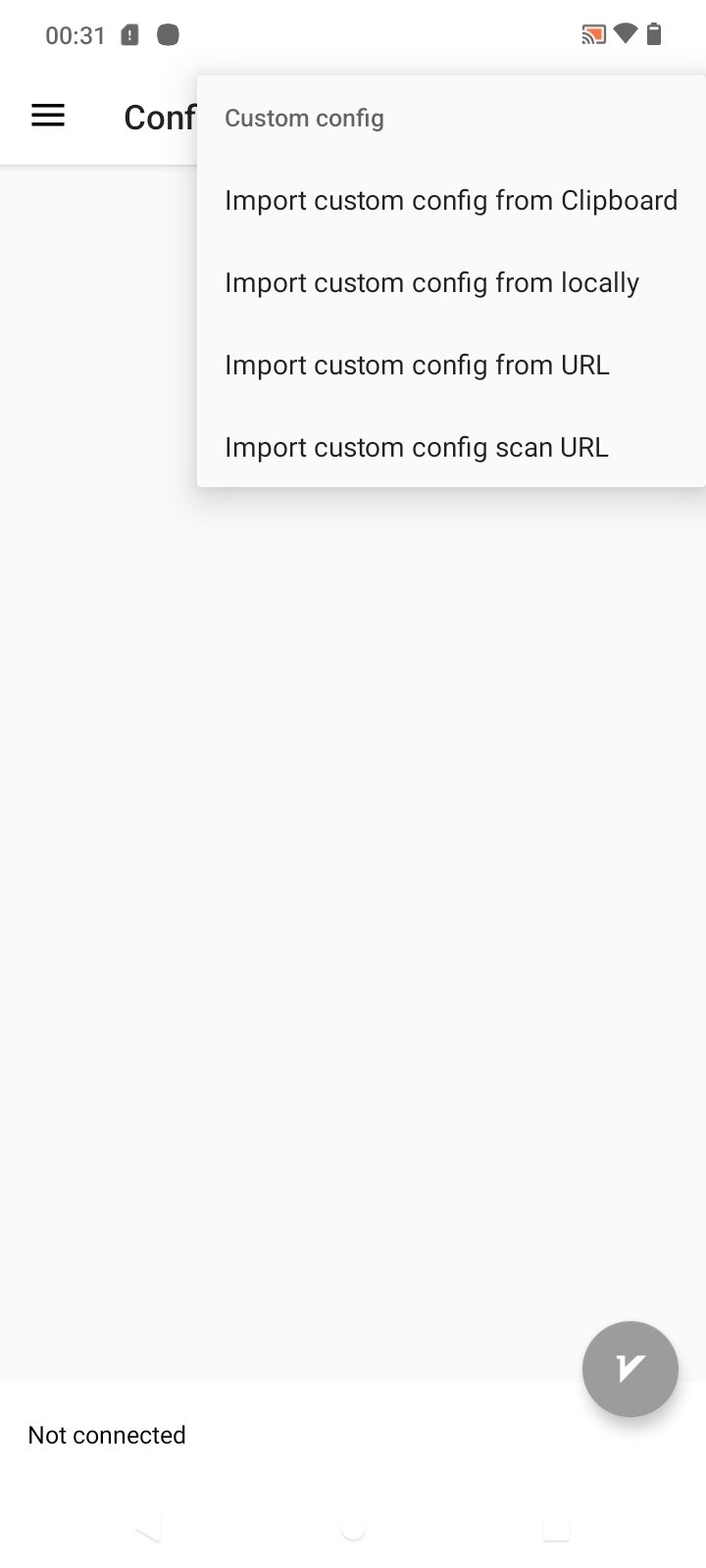A small, detailed image from a website shows a complex configuration popup. The top of the image displays a timestamp of 0.31 seconds, with Wi-Fi enabled and the battery at approximately 80% capacity. On the left side, there is a partially visible menu bar with an entry labeled "CON," likely abbreviated from "CONFIGURATION," obscured by a popup window titled "CUSTOM CONFIG." This popup presents several options: "IMPORT CUSTOM CONFIG FROM CLIPBOARD," "IMPORT CUSTOM CONFIG FROM LOCALLY," "IMPORT CUSTOM CONFIG FROM URL," and "IMPORT CUSTOM CONFIG SCAN URL." A grey circle with a white checkmark symbol is also visible. At the bottom-left corner of the popup, the status indicates "NOT CONNECTED." The image is compact, conveying limited but crucial information related to custom configuration and connectivity settings.